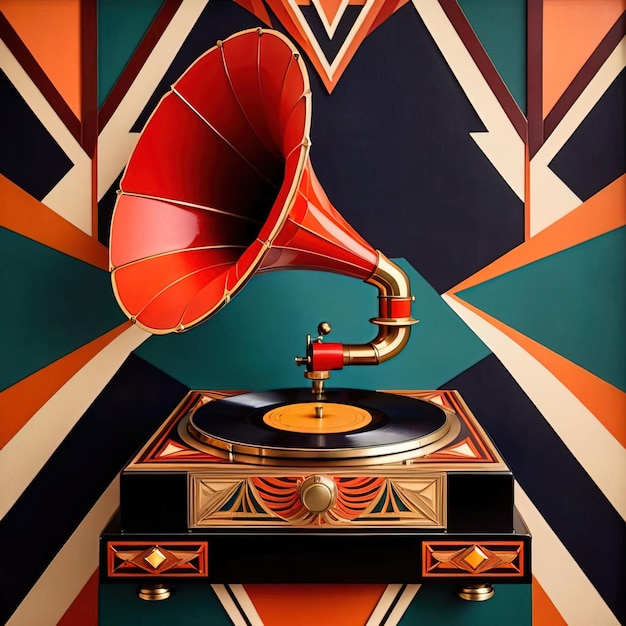This image showcases an ornate phonograph set against a striking, geometric background that evokes an art deco aesthetic. The backdrop is composed of angular, vector graphic shapes in dark blue, white, orange, reds, and turquoise, creating the illusion of a mountainous landscape. At the center of the scene sits a vintage phonograph with a burnished bronze body adorned with intricate orange and blue accents. Notably, it features a prominent red horn speaker with golden rim lining, made of bronze or gold-colored metal, which dramatically flares outward above the turntable. The phonograph is poised with a vinyl record that has an orange label at its center, adding to the overall vibrant and visually stimulating composition. The image is devoid of any text, allowing the detailed design elements to stand out.